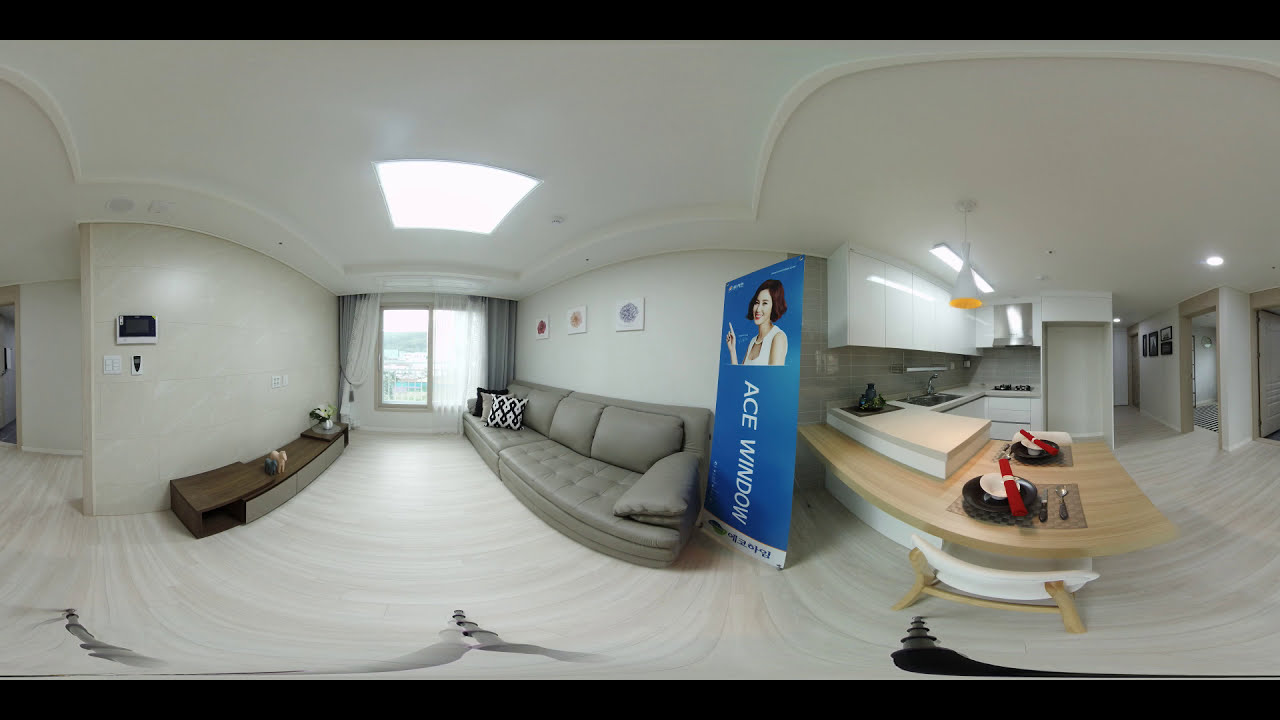This image presents the interior of an apartment with a fisheye lens effect, creating a curved visual distortion. The room is predominantly decorated in varying shades of gray. In the center of the scene, there is a large blue vertical banner with white text that reads "Ace Window." The banner features a woman in a sleeveless white dress with chin-length dark hair pointing upwards.

To the left of the banner, a gray couch adorned with black, white, and gray pillows sits near a window adorned with sheer and gray draperies. Directly across from the couch, a wooden console table holds a decorative floral arrangement. A large rectangular light fixture hangs from the ceiling of the living room.

Moving right from the living room, one enters the kitchen area. The kitchen is compact, featuring a counter with plates, knives, and forks, a sink, and a small stove, against a backdrop of white and light gray hues. Notably, the kitchen lacks a refrigerator, adding an unconventional touch to the scene.

Farther right, there's a hallway leading to other rooms. The floor throughout the apartment, including the kitchen, is gray. In one of the background rooms, a black and white checkerboard floor is visible, suggesting another design element consistent with the apartment's color theme. The view out of the large window reveals a cityscape with distant mountains and buildings, emphasizing the apartment's urban setting.